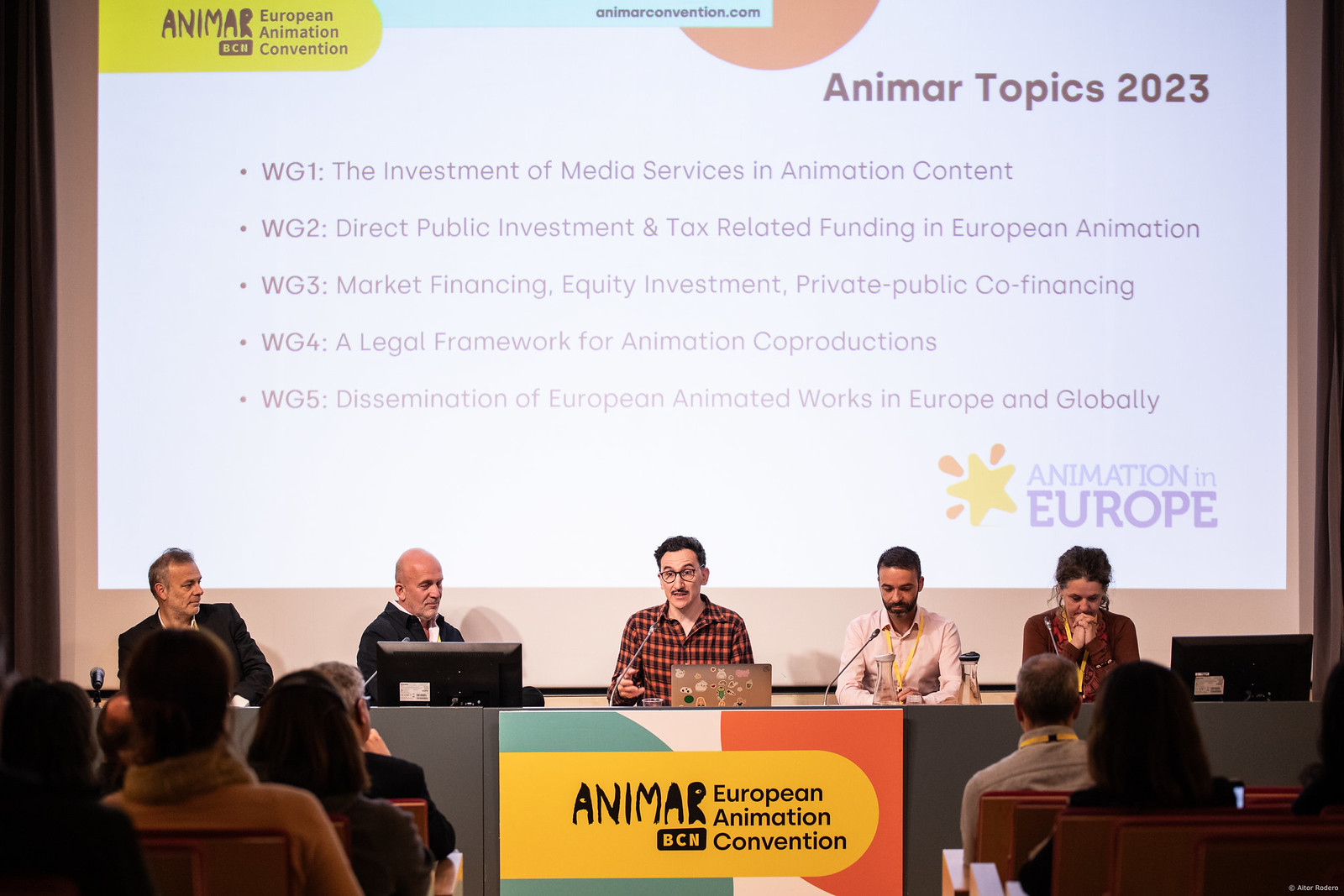This rectangular photograph captures a panel discussion at the Animar European Animation Convention. The image shows five individuals seated at the front of the panel facing a seated audience. At the center of the panel is a man with dark hair and glasses, wearing a plaid shirt, currently speaking to the audience. To his left sits a bald gentleman in a black suit with a white shirt and next to him, on the far left, is another man in a black jacket and white shirt with salt-and-pepper hair. To the speaker's right is a man with dark hair and a mustache, dressed in a light pink shirt. On the far right end of the panel sits a woman in a reddish-colored shirt, her dark hair contrasting with her attire, and she is leaning forward with her hands crossed.

The panel is seated behind a desk or table with a sign displaying "Animar European Animation Convention." Behind them, a screen projects information indicating "Animar Topics 2023." The screen lists various discussion topics: WG1, the investment of media services and animation content; WG2, direct public investment and tax-related funding in European animation; WG3, market financing, equity investment, private-public co-financing; WG4, a legal framework for animation co-productions; and WG5, dissemination of European animated works in Europe and globally.

Colors popping in this image include yellow, green, red, purple, and light blue, adding vibrant details to the scene. In the foreground, on either bottom corner of the photograph, audience members can be seen, indicating an engaged crowd.